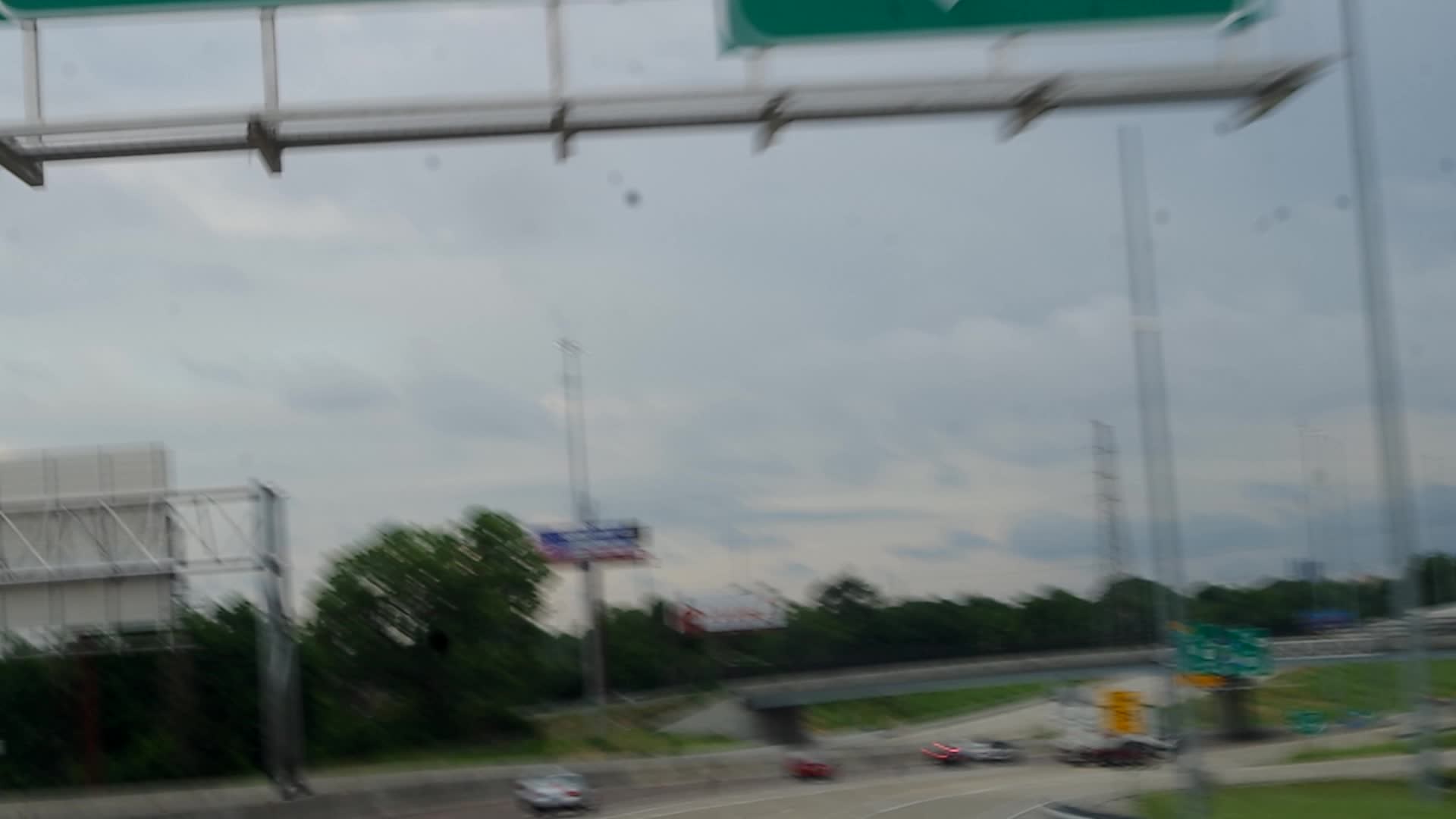This image depicts a blurry highway scene taken from an elevated or aerial perspective. At the bottom of the image, the highway features about four or five blurred cars, including a gray or red car with its taillights on, and a couple of white ones. The cars are approaching an overpass positioned in the bottom center of the frame. On the right, a visible off-ramp leads to a patch of green grass, surrounded by the border of green trees that line the highway.

Above the roadway, two green signs attached to lattice structures stretch across the road, visible only in part due to the blur. The sign on the left is oriented for oncoming traffic, which is not visible in the frame. There are four tall poles scattered throughout, one displaying a blue, white, and red board, although the text is illegible. Additionally, there are telephone or electronic wires visible in the distance. The sky is overcast and cloudy, with a bit of light seeping through, adding to the overall haziness of the image.